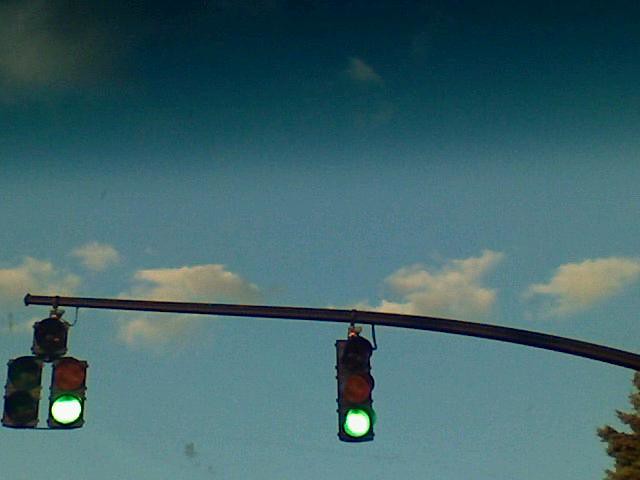The image captures a moment at an intersection, where we're looking up at two sets of traffic lights hanging from a long, dark gray pole. The left light, which is designed for a turning lane, has five bulbs but only its green light is illuminated. The right light, which controls a regular single lane, also shows a lit green signal. The background sky is a gradient of dark to lighter blue, peppered with a few broken clouds stretching from left to right across the middle; a larger cloud sits at the top. The scene seems to have been taken through a slightly tinted windshield, adding a perceived older and grainier look to the photo, possibly with some stains. This suggests the picture might have been snapped hastily, potentially while the car was stopped at the light which then turned green. In the bottom right corner, a portion of a tree is visible, contributing a touch of natural greenery to the composition. The overall lighting and color indicate it is daytime, albeit a part of the day when the sky can appear darker, adding a nuanced atmosphere to the photograph.